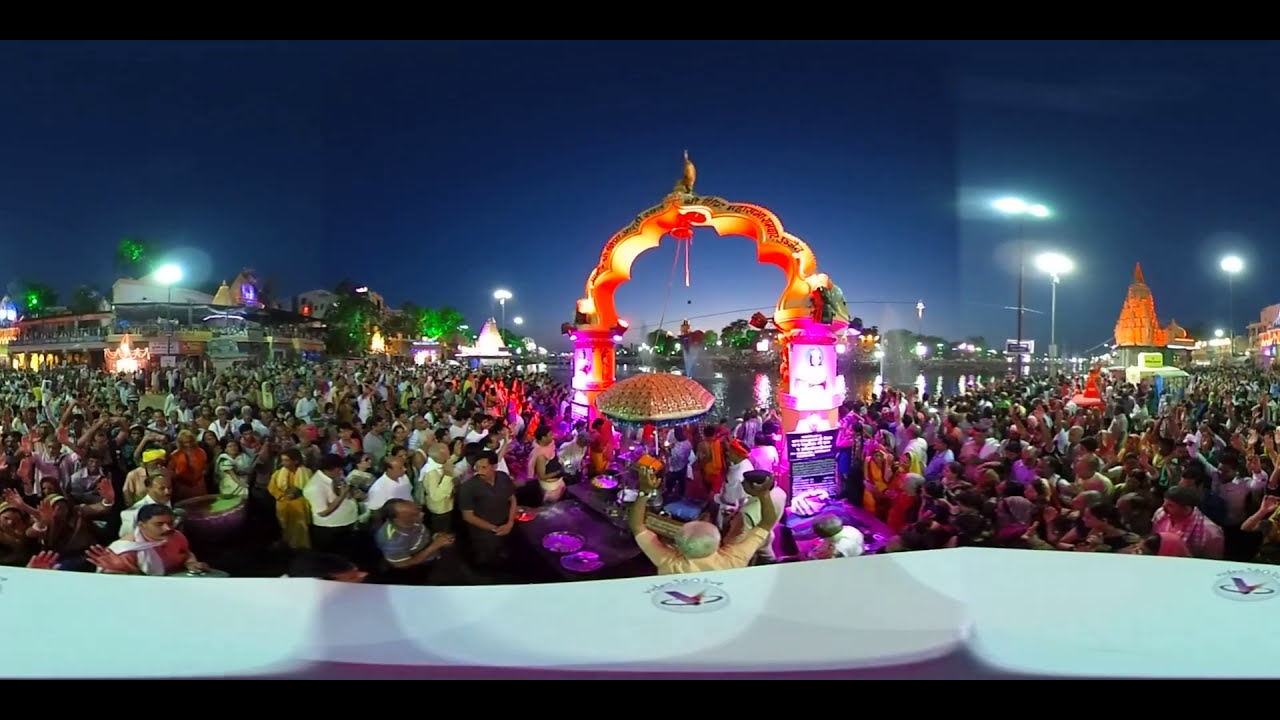The photograph depicts an outdoor nighttime scene, possibly a music festival, given the large crowd tightly packed together. Central to the image is a golden illuminated arch adorned with pink, orange, and white neon lights. Beneath the arch, there is a stage with a golden umbrella, and a person can be seen with both arms raised in the air. The crowd predominantly appears to be of Indian descent, with some individuals on the left side waving their hands towards the camera. The sky transitions from a deep blue at the top, indicative of late dusk, to the remaining traces of sunlight on the horizon. A building in the background has lights reflecting off nearby water, enhancing the scene's vibrant colors, which include shades of orange, pink, purple, white, green, and blue. The photo also features some visible imperfections, possibly from stitching multiple images together, noticeable by color changes and a faint line through the image. At the very bottom, there is a white area with a logo or writing that is not fully legible, suggesting the photograph might have been taken from a higher vantage point, perhaps over a stage or shelf.